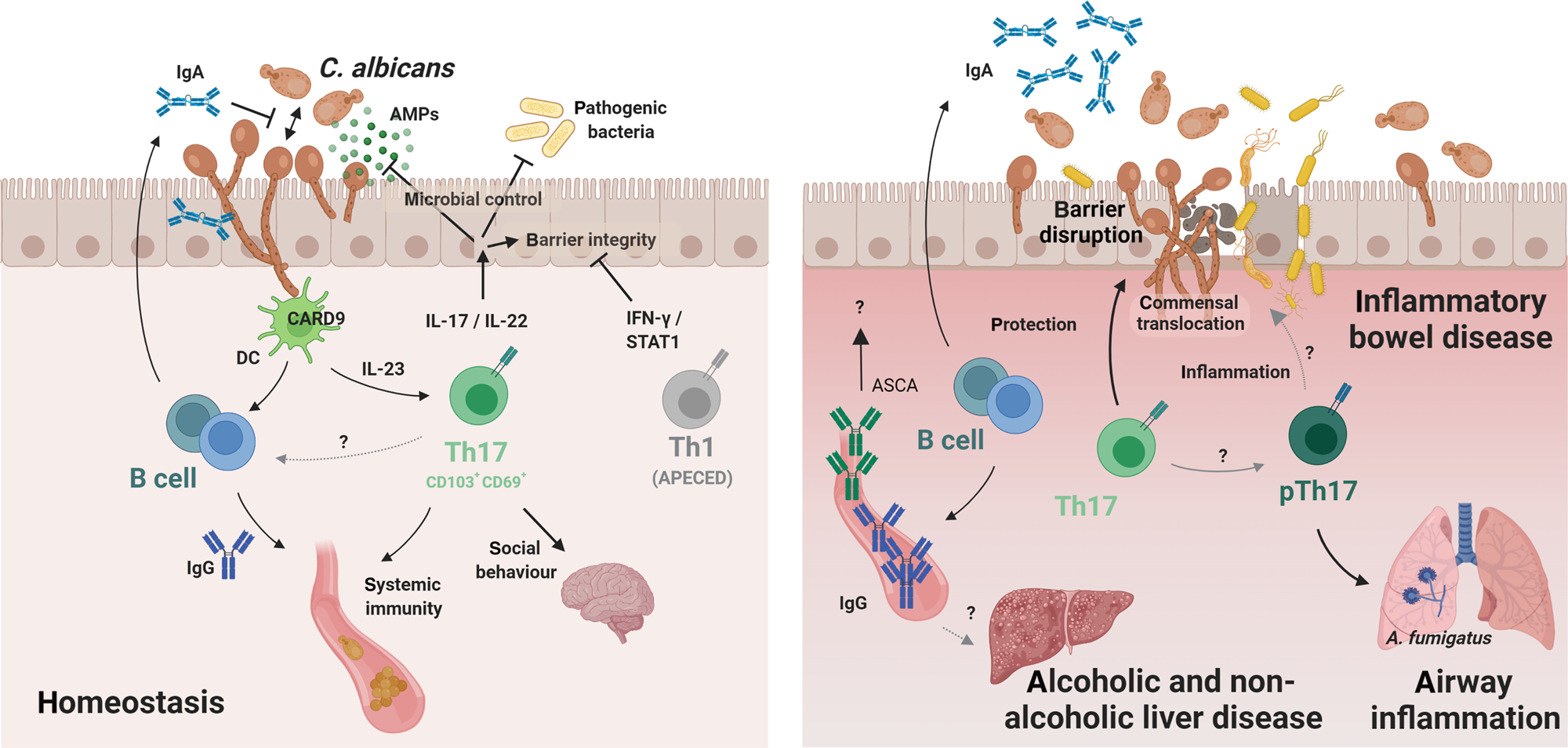The image features a detailed medical diagram with a white background, divided into two parts. The left section is primarily light pink and includes multiple illustrations and labels. It showcases components related to C. albicans pathogenic bacteria and an array of cells like B cells and TH17. Important terms mentioned here include homeostasis, microbial control, barrier integrity, IL-17, IL-22, IL-23, systematic immunity, and social behavior as it relates to the human brain. This side of the image also displays various shapes and colors, such as blue circles, a green circle, gray circle, brown circles with long threads, and yellow capsule-like structures.

The right section transitions from light to dark pink and discusses medical issues like inflammatory bowel disease, airway inflammation, and both alcoholic and non-alcoholic liver disease. It also highlights terms such as barrier disruption, protection, chromosomal translocation, and inflammation. Visual elements in this part include illustrations of a liver, lungs, circles in different colors (dark and light green, blue, teal), and various bacterial representations like yellow spiky bacteria. Both parts combine to provide a comprehensive depiction of the interactions between microbiota, immune responses, and chronic diseases.